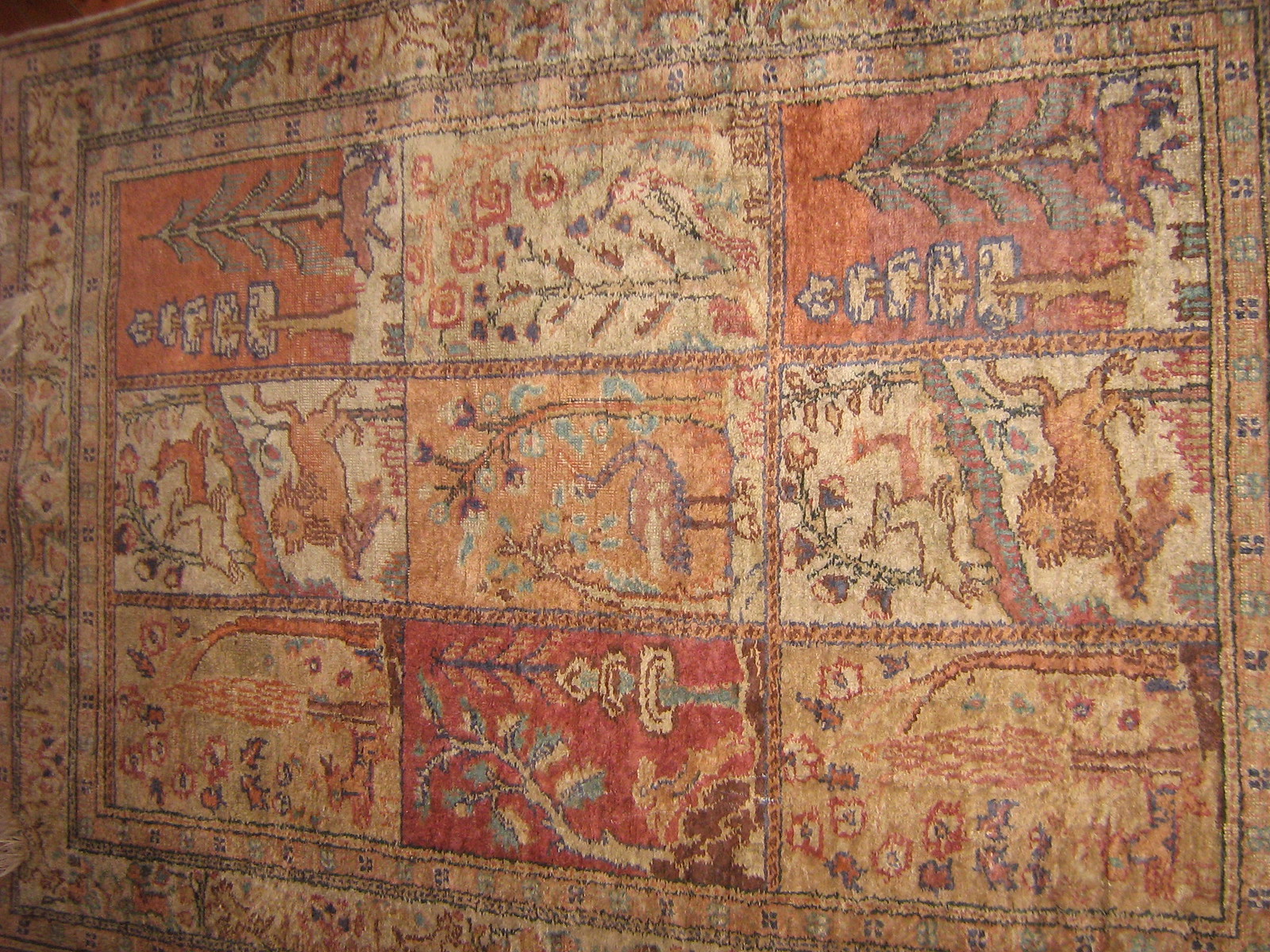This photograph displays a large, intricately patterned area rug, likely around six feet across, laid out on a wooden floor. The rug features a 3x3 grid of rectangular panels, each depicting a unique scene, framed by detailed floral borders and various intricate patterns. Dominant colors include shades of orange, beige, bluish-gray, and brown-orange. 

Most panels prominently feature trees, some with animals. Specific images include a tall evergreen tree with a signpost, a lion with prey, a deer, a peacock beside a tree, a fountain, and a rabbit amidst trees. Repeating designs are noted, such as a person standing with birds in a tree-trunk scene and deer running by a tree, each appearing twice. Detailed handcrafted weaving suggests a high level of artisan skill, especially evident in the floral borders and repetitive nature motifs around the central images.